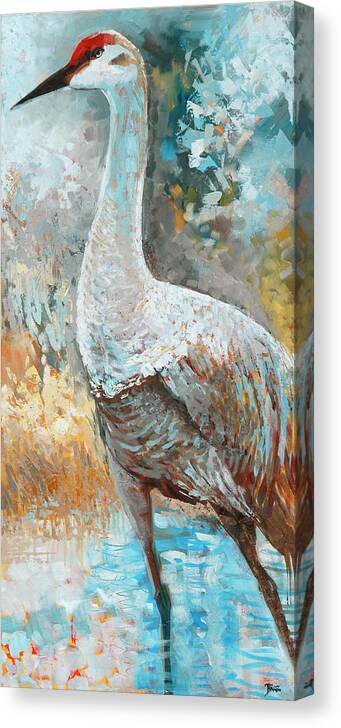This is a tall, narrow painting, approximately with a 5 by 16 aspect ratio, depicting a heron. The heron occupies the entire canvas, from its thin legs standing in water at the bottom, up to its head adorned with a red crest and a black beak at the top. Painted in oil, the heron itself is mostly white, with details of brown and blue accents that add depth and dimension. The bird's neck is notably white with hints of blue and brown, while its feathers darken to brown and orange hues. The impressionistic background features an abstract mix of blue, green, white, and yellow colors, representing water, reeds, and clouds, though not clearly defined. The overall scene is a close-up portrait of the heron facing left, its black eyes adding to the lifelike portrayal amidst the swirling colors.